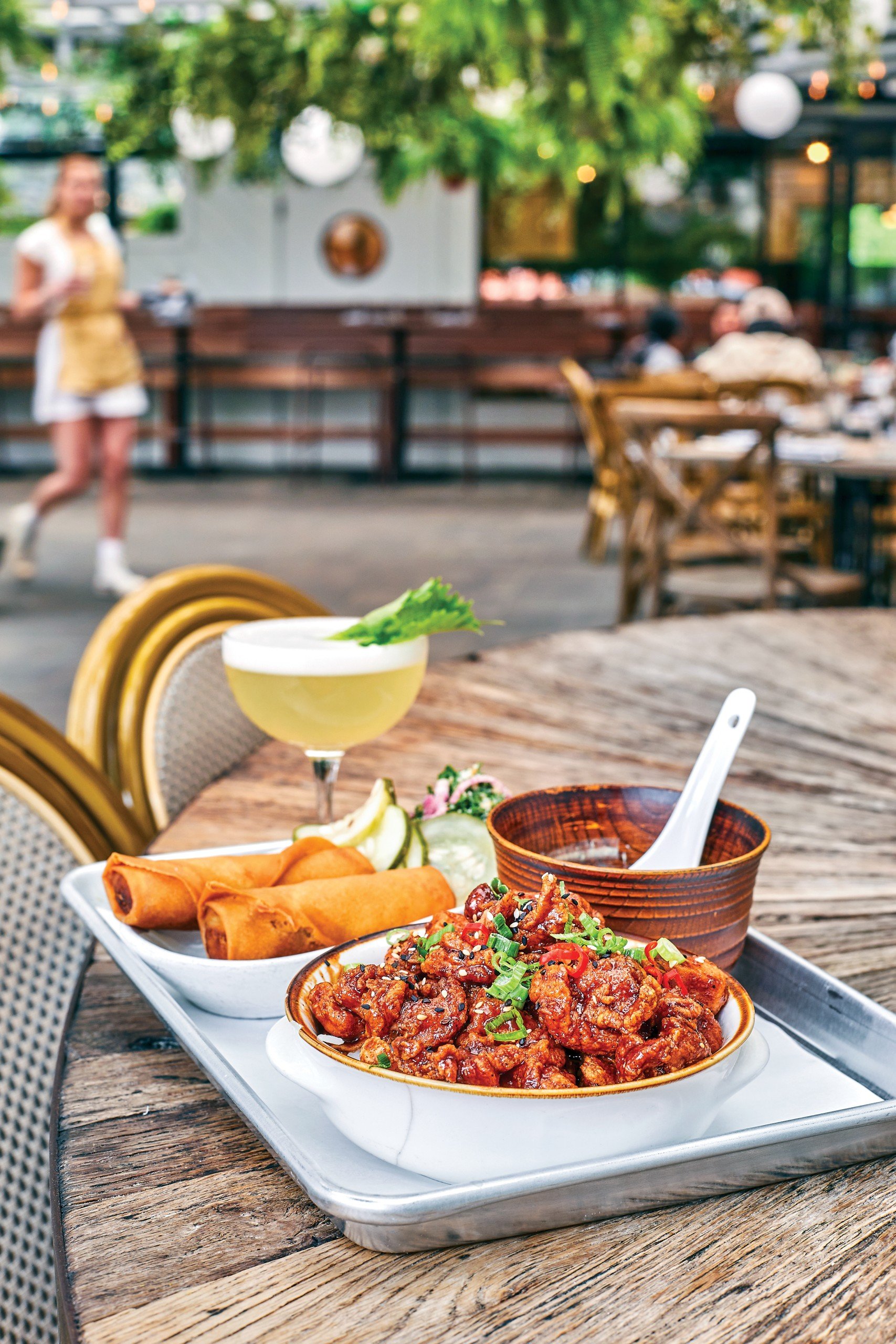This image captures an inviting outdoor patio area of a rustic-style restaurant, bathed in natural light streaming from above. The scene centers around a brown, wooden table, only partially visible, adorned with an assortment of tantalizing food items and a drink. Dominating the table is a silver-colored tray, used as a serving platter, on which various bowls are placed. 

A white bowl is filled with a vibrant stir-fry, possibly teriyaki chicken or shrimp, smothered in a savory sauce and garnished with green scallions, sesame seeds, and some mixed vegetables including green leaves and tomatoes. Another white bowl holds a pair of golden-brown egg rolls, and nestled next to them appears to be slices of apple, adding a fresh contrast. 

In addition, there's a brown bowl containing what looks to be a communal dish, equipped with a white ladle for serving. On the side of the table, a refreshing margarita with a yellow-green hue is placed, garnished with a green leaf. 

Adding to the lively atmosphere, a waitress is visible to the left, diligently carrying food items. The surrounding ambiance is enhanced by lush greenery with leaves hanging around the space, creating a harmonious blend of indoor comfort and outdoor freshness.